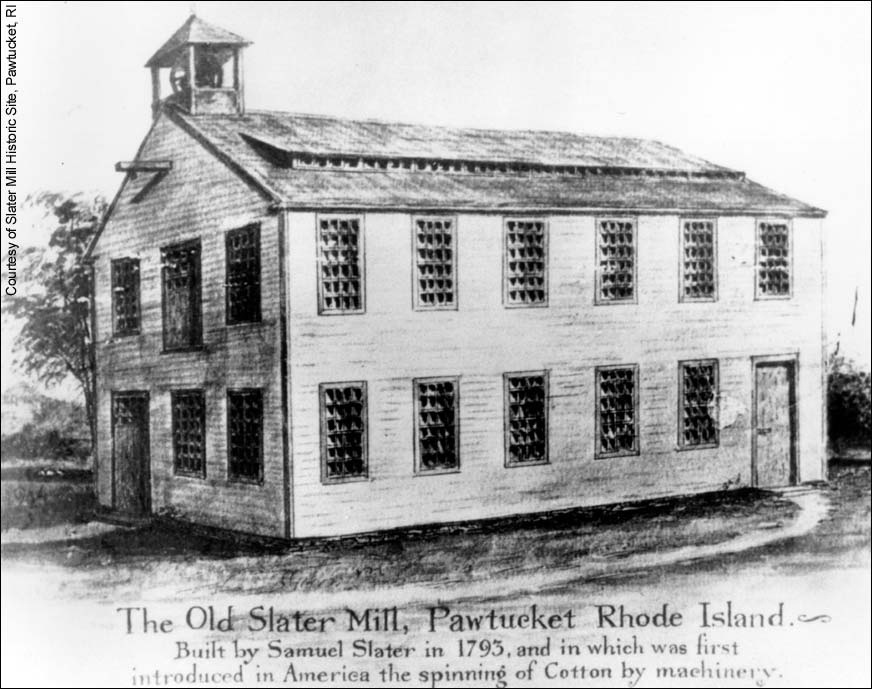The image is an intricate artist's rendition of the Old Slater Mill in Pawtucket, Rhode Island, built by Samuel Slater in 1793. This historic cotton mill, where the spinning of cotton by machinery was first introduced in America, is depicted as a two-story oblong building with numerous windows. The front façade features five windows on the ground floor, with a door beneath the third window from the left, and six windows on the upper level. The structure has a bell turret atop the roof's peak, with a visible object inside, potentially a bell. The mill, drawn possibly with graphite pencil, is surrounded by shrubbery, grass, and trees. The paper is white, enhancing the detailed, old-schoolhouse appearance of the building. The image is courtesy of the Slater Mill Historic Site in Pawtucket, Rhode Island, as noted along the left border.